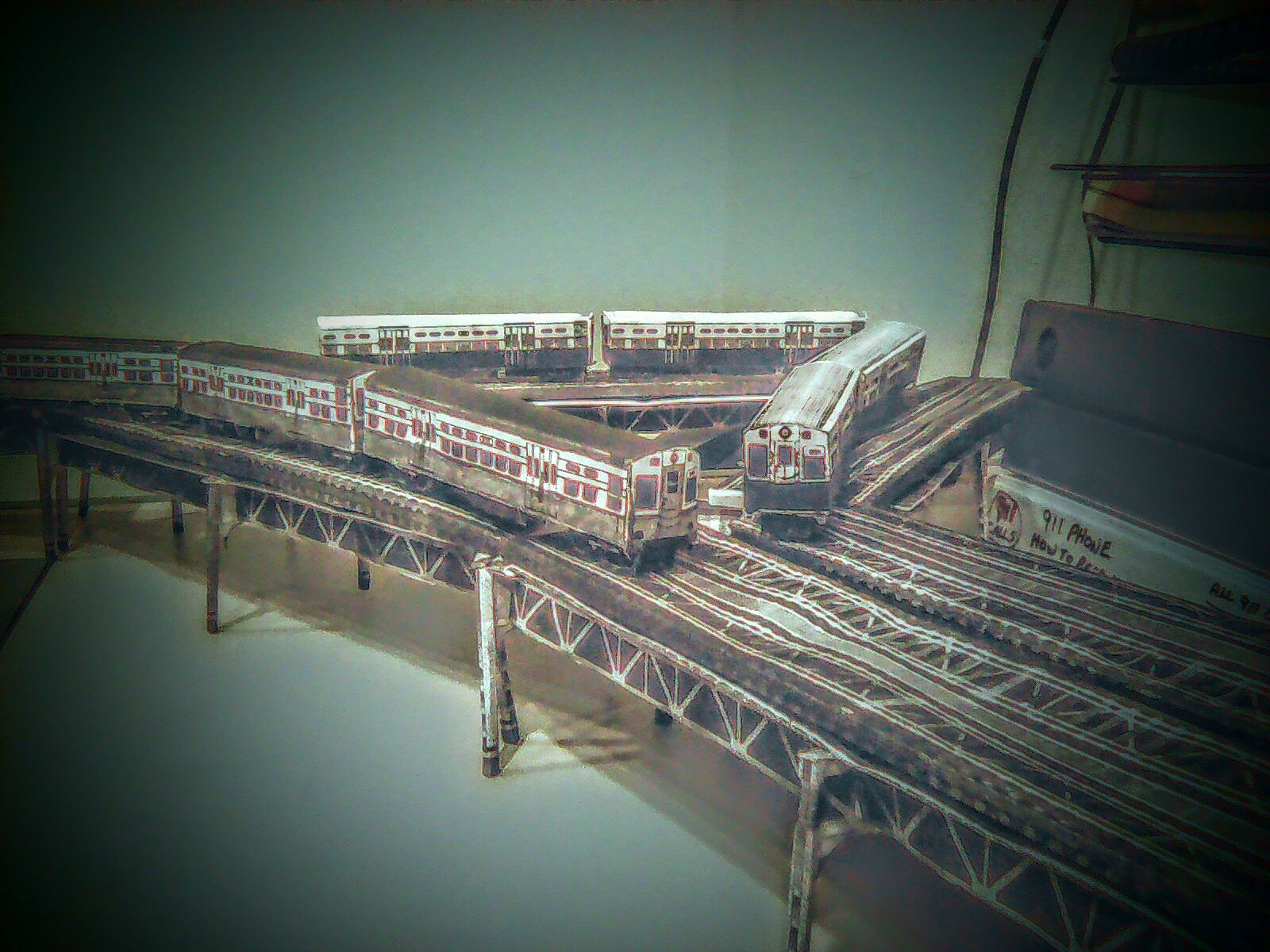This image depicts a meticulously crafted 3D model of an elevated subway system, resembling those found in New York or Chicago. The model consists of small tin train carriages, each approximately 12 inches long, 2 inches wide, and 3 inches high, set on an elevated track structure. 

The track originates from the bottom right corner and splits about halfway across the image into a Y shape. These Y sections guide the trains along different paths, eventually forming a triangular intersection where three separate train carriages converge. Two of the carriages are advancing towards this triangular junction, while the third carriage is situated on an additional interconnected track within the triangle. 

The trains are designed in monochromatic tones of white, black, and gray, accented by red trim around their windows, and they stand on a network of legs above what appears to be a body of water. The background of the image features a grey-white overcast sky. Intriguingly, there is a faint figure that resembles a boat in the top right corner, adding depth and mystery to the scene. In juxtaposition with this intricate set, some three-ring binders are placed for scale, highlighting the miniature but detailed construction of the artwork.